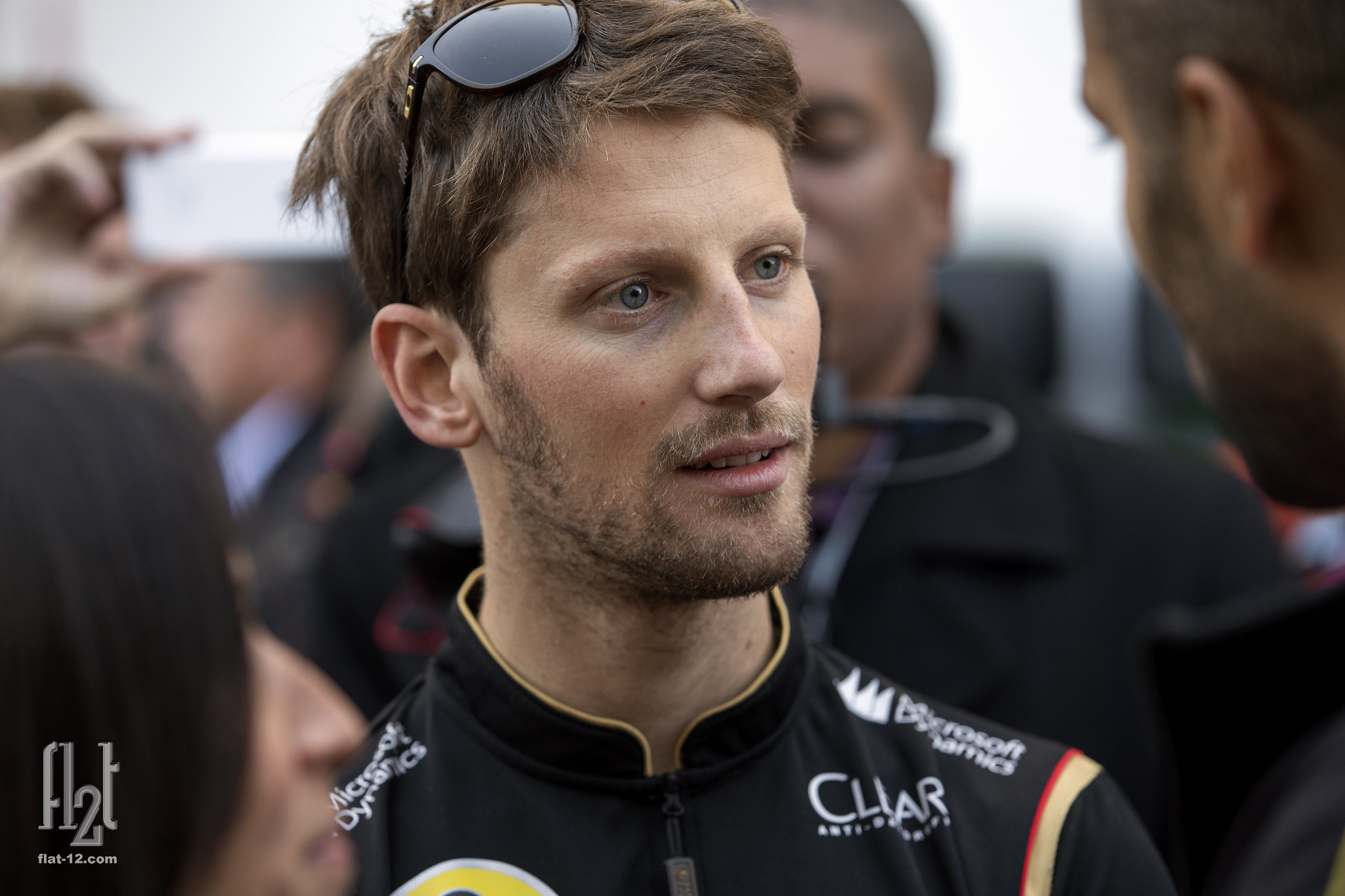This wide rectangular photograph captures a mid-twenties race car driver from the shoulders up, positioned in the center with his head slightly tilted to the right. He has thick, short brown hair, and light blue eyes that gaze to the right, partially obscured by thick brown eyebrows. He sports a short brown beard and mustache, and black sunglasses rest atop his head. He is dressed in a black zip-up racing uniform adorned with various logos in white font, featuring a yellow and red streak on his right bicep. Surrounding him are blurred figures in the background, giving the impression of an interview setting. On the bottom left, a woman's blurry profile with brown hair can be seen, while in the top right corner, a man with light brown skin and darker stubble looks towards the main subject. Notably, the bottom left corner of the photo reads "FL2T, flat-12.com" in silver font.